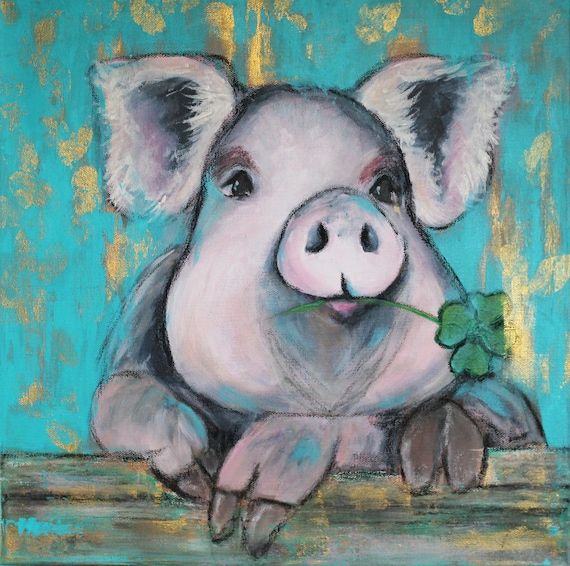This is a detailed painting, likely on canvas, depicting a pig against a turquoise background with gold and cream-colored splotches. The pig, rendered in a painterly and almost sketched style, features a gourd-shaped face, big expressive eyes, and a small pink mouth holding a green four-leaf clover on a long stem. The pig’s fur appears whitish gray with hints of pink and turquoise, the same shade as the background, blending softly with no strong outlines. The pig has dark spots, particularly inside its furry ears, and appears to lean on or sit atop a wooden plank or fence with three visible hooves resting on it. The details create a whimsically detailed and somewhat feminine portrayal of the pig, characterized by its soft, undefined lines and mixed colors.